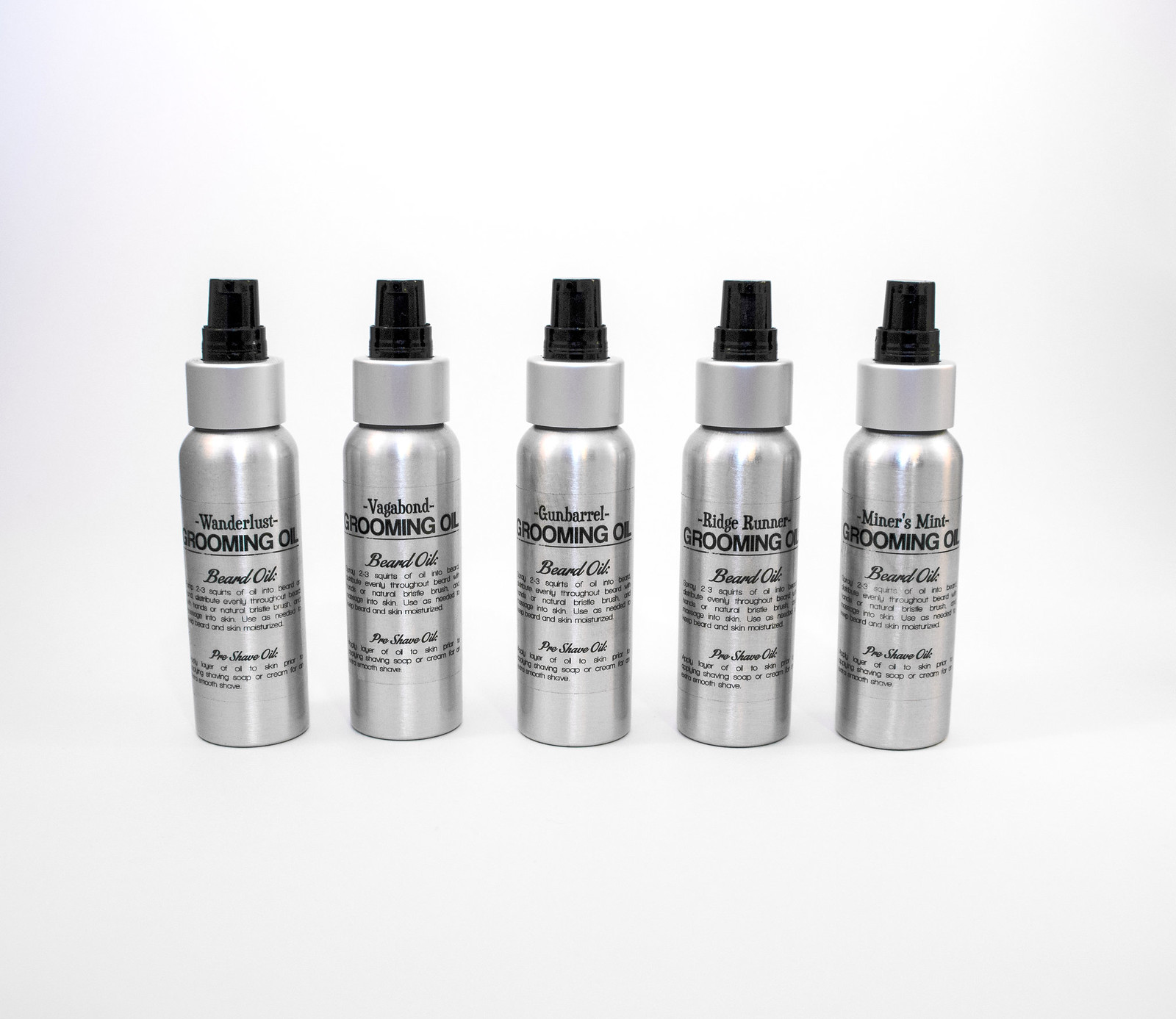The image features a close-up, indoor color photograph showcasing five small cylindrical spray bottles of beard oil on a white surface with a white background. Each bottle is silver metallic with a black spray dispenser secured by a silver cap. The labels of the bottles have black printing, prominently displaying "GROOMING OIL" in capital letters. Below this, in cursive writing, each label indicates "Beard Oil." The five bottles, from left to right, are labeled with different scent names: Wanderlust, Vagabond, Gun Barrel, Ridge Runner, and Miner's Mint. Additionally, there's a mention of "pre-shave oil" on the labels. Despite slight variations in scent names, the layout and other text on each bottle remain consistent. The overall image is in sharp focus, clearly displaying the product details, although some smaller text remains too tiny to read.